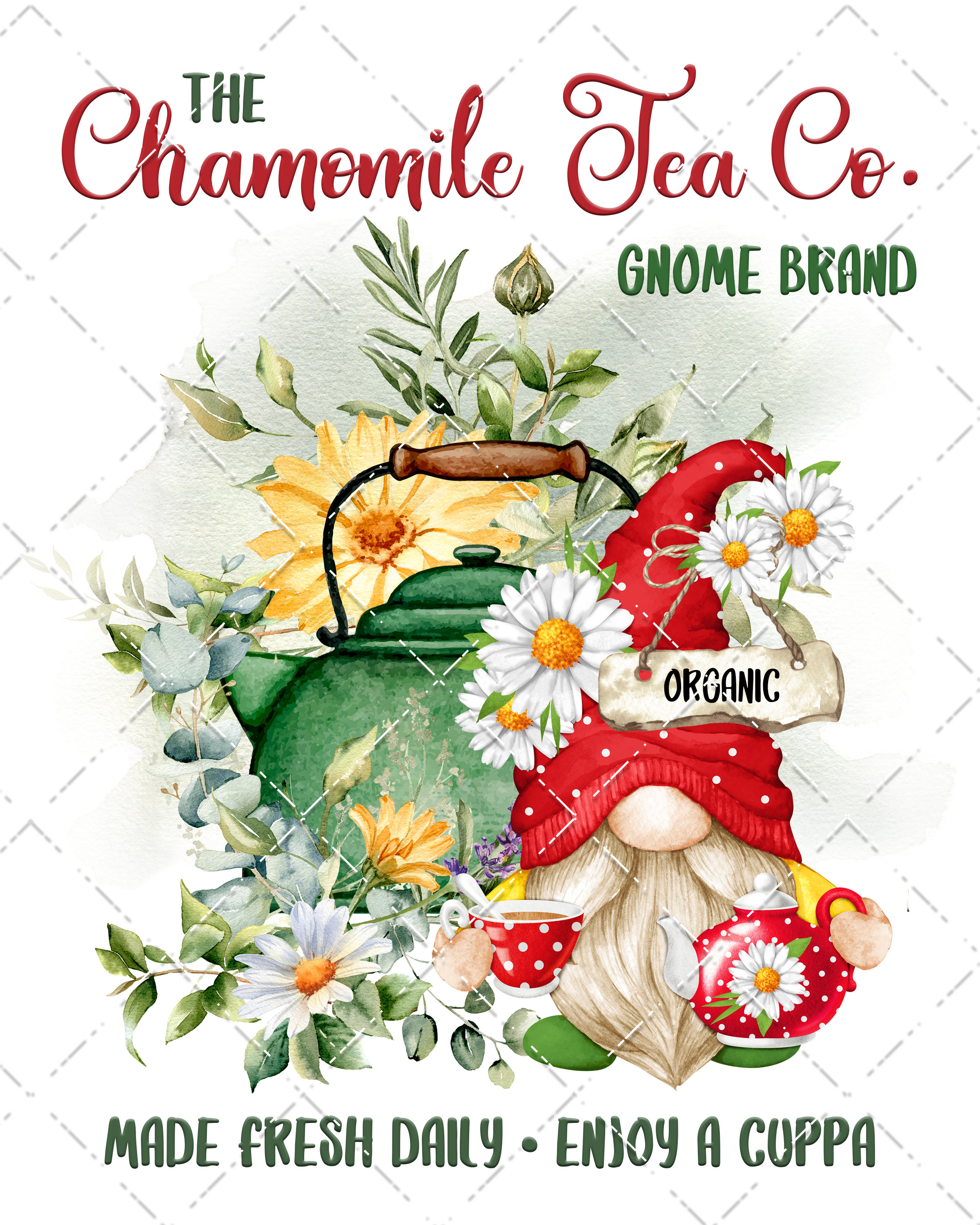The image is a colorful advertisement featuring an intricate design centered around a gnome and a green teakettle. At the top, elegant script text reads "The Chamomile Tea Company" with "Gnome Brand" highlighted in green. Below this, in smaller green text, it says "Made Fresh Daily. Enjoy a cuppa." The centerpiece shows a charming gnome with a white mustache and beard, wearing a red hat adorned with daisies and a sign reading "organic." The gnome holds a red teapot and a matching red cup with white polka dots, which have flowers on them. Behind him is a green teakettle with a prominent yellow flower, surrounded by various greenery and flowers. The entire scene is overlaid with a delicate windowpane-like diamond pattern.